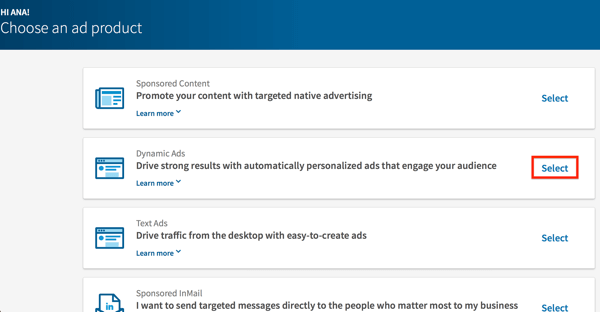Screenshot of a LinkedIn Ad Management Interface:

The top of the interface features a blue bar with "HiAnna" displayed in the top left corner. Below that, there are multiple sections in a rectangular layout. The first section is titled "Sponsor Content" with a description underneath that reads, "Promote your content with targeted native advertising." This section has a blue "Select" button.

The second section is labeled "Create Dynamic Ads" in black text, accompanied by a note stating, "Drive strong results with automatically personalized ads that engage your audience." This section is outlined with a red border and also has a blue "Done" button.

The third section, titled "Text Ads," states, "Drive traffic from the desktop with easy to create ads," and includes options to "Learn More" and "Select." 

The fourth section has grey text reading "Sponsored Email," with black text stating, "I want to send targeted messages directly to the people that matter most to my business," accompanied by a "Select" button.

The background of the interface is white, with a shadow effect under each of the four sections. The entire interface appears to be a LinkedIn document window.